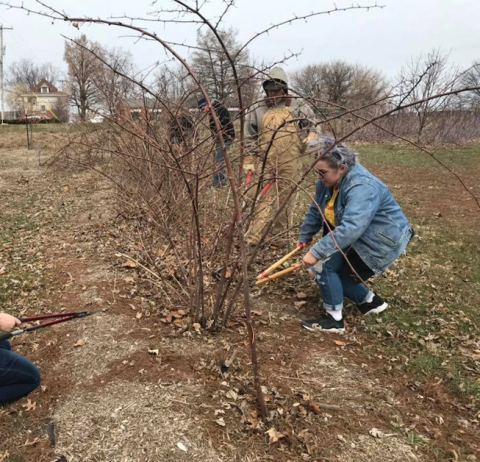The image captures an outdoor scene of several individuals pruning rows of thin trees. Central to the photo is a woman dressed in outdoor work attire, including jeans and overalls, who is using lopping shears to trim branches. She is crouching down and focused on her task. Visible to her side, another person, also in work clothes—a denim jacket, yellow shirt, jeans, and black sneakers—holds yellow clippers, poised to prune another branch. In the background, additional people are engaged in similar activities, one notably in tan overalls with a hoodie, standing at full height, and others dressed in darker clothing. The scene is set against a backdrop of houses visible in the distance under an overcast, whitish-gray sky. The color palette primarily features earthy tones of brown and muddy green, characteristic of the season, with green grass and scattered leaves on the ground. The composition is bright and clear, indicative of ample natural lighting. The photo is square in format, capturing the rustic and industrious atmosphere of a tree-pruning session.